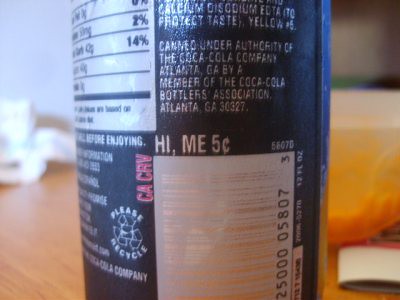This close-up photograph captures a portion of the back side of a Coca-Cola product can, predominantly dark midnight blue, with a combination of black and white panels featuring silver lettering. The image reveals a segment of the nutritional label showing only partial values (2% and 14%), and the list of ingredients, which includes calcium disodium EDTA to protect taste, and yellow number 5 or 6. The can bears the inscription "canned under authority of the Coca-Cola Company, Atlanta, Georgia" by an associated bottler. The lower left corner includes fine print mentioning recycling information and a 5-cent deposit return for Hawaii and Maine. Additionally, the bottom right corner displays a scannable UPC code in white. The can is positioned on a wooden table, with Tupperware visible in the background, suggesting a kitchen setting during daylight hours.